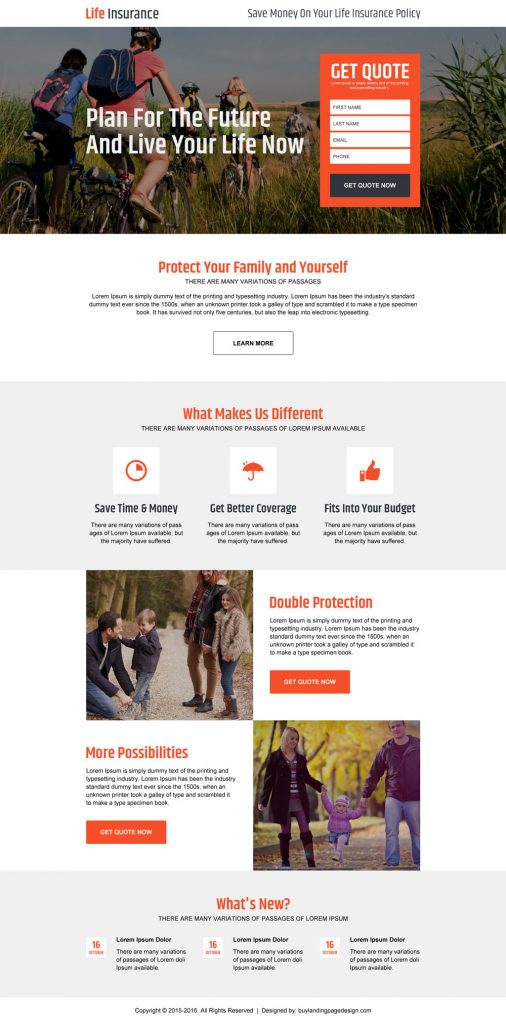Homepage of the Life Insurance Website:

The homepage for the Life Insurance website prominently features its motto, "Save money on your life insurance policy." Beneath this tagline is a vibrant stock image banner depicting a group of people biking through a tall grassy field on a bright, sunny day. Superimposed over the banner is another motivational slogan, "Plan for the future and live your life now," adding to the site's inviting atmosphere.

To help users get started, there's a "Get Quotes" box where visitors can enter their first name, last name, email, and phone number for more personalized information. 

Below this section, the homepage provides a wealth of information paired with basic icons and stock images, contributing to a friendly and reassuring aesthetic. These include:
- "Protect your family and yourself”
- "What makes us different"
- "Double protection"
- "More possibilities"
- "What's new"

All of the accompanying stock images showcase families and parents enjoying quality time with their children in various nature settings, reinforcing the theme of security and happiness.

Under the "What makes us different" section, icons illustrate key features:
- "Save time and money" represented by a graph
- "Get better coverage" symbolized by an umbrella
- "Fits into your budget" depicted by hands giving a thumbs up

Finally, the "What's new" section lists several dates, though currently, it features placeholder text ({}) indicating that fresh content will be added soon.

Overall, the homepage combines engaging visuals with clear, actionable information, inviting users to explore more about their life insurance options.